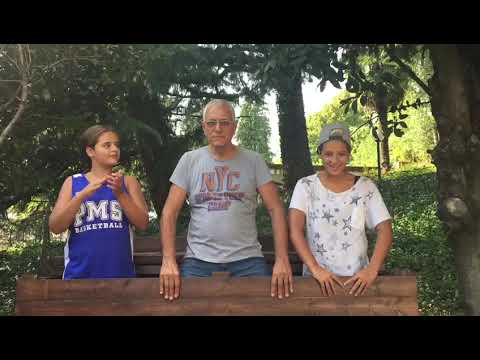In the image, an elderly man stands in the center, flanked by two teenagers, each around 13-14 years old. The man is wearing glasses and has thinning silver hair. He’s dressed in a gray t-shirt with the letters "NYC" in light orange at the top and some smaller, partially obscured text below. His blue jeans are partially visible as he grasps a dark brown wooden bench in front of him, his fingers curled over the top. 

To his left stands a teenage girl in a blue basketball tank top with "PMS Basketball" written on it in large white letters. Her hands are together as if clapping, and she’s looking at the man with a smirk on her face. On his right, another teenager wearing a white short-sleeved shirt adorned with black and gray stars stands with both hands holding the bench. She also wears a backwards gray baseball cap. 

All three individuals are positioned in front of what appears to be a wooden bench or gate, set against a backdrop of a lush forest with both deciduous and fir trees. Some of these trees are lit up in the distance, suggesting they might be near the end or side of a path. The scene captures a moment of the trio posing for a photograph amidst the natural greenery.